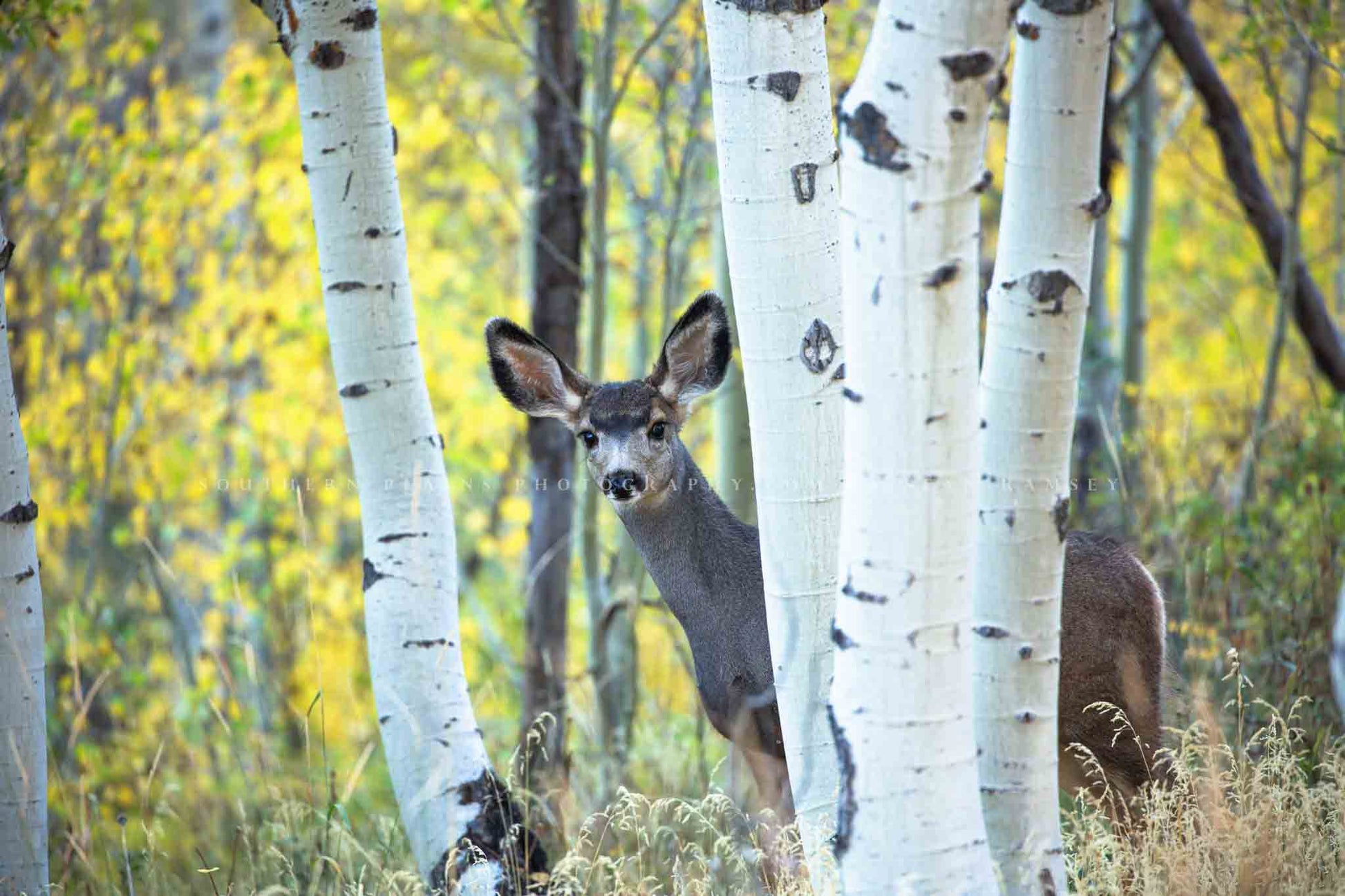A captivating photograph captures a curious deer, standing amidst a serene woodland setting and gazing directly into the camera lens. The deer, neither a juvenile nor fully grown, boasts a medium size with no antlers and notably large ears perked attentively. Its head and neck, along with one front leg, emerge from between two slender trees with striking white bark, giving the impression that the deer is playfully peeking through the natural gap. Behind the trees, the deer's rear end is visible, completing the intriguing partial view of its body. The background reveals an array of trees adorned with vibrant yellow foliage, creating a picturesque autumnal scene. In the foreground, delicate, wheat-colored grasses sway gently, adding texture and depth to this tranquil, nature-filled composition.